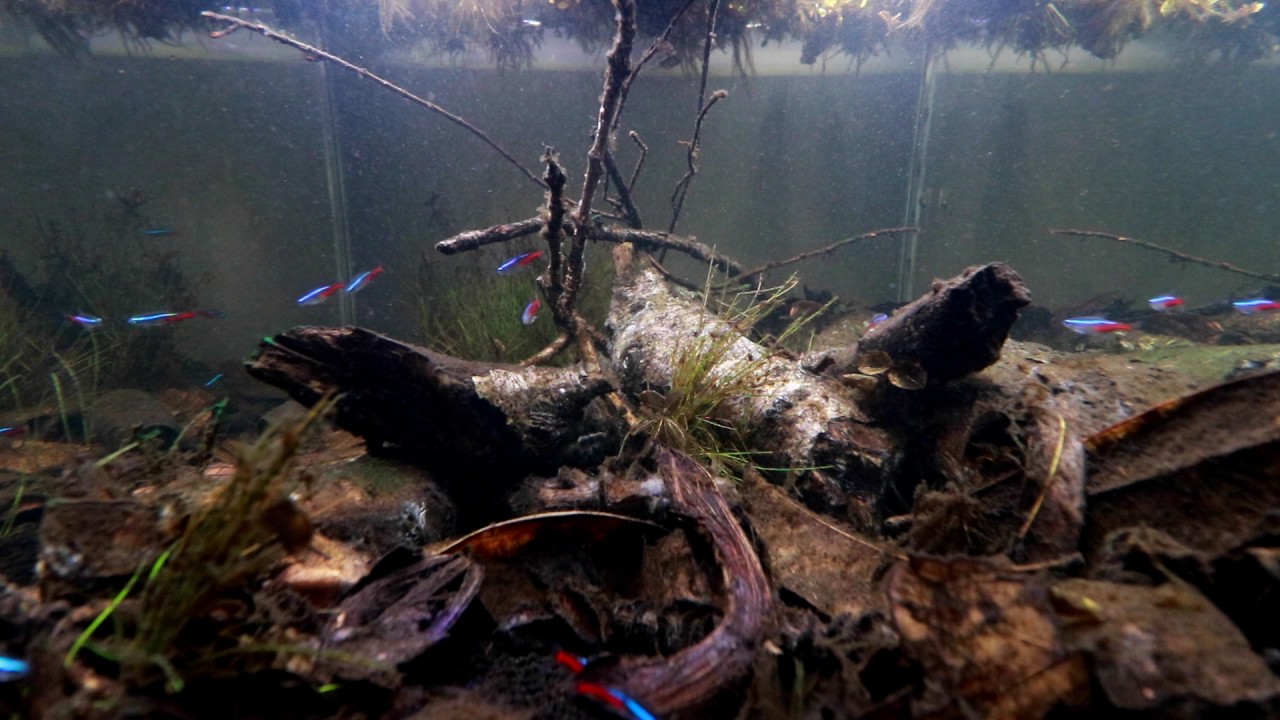This photograph captures an underwater view of a large tank or aquarium, teeming with aquatic life and natural elements. The tank is filled with various logs, sticks, grasses, and water plants, with a hint of seaweed adding to the natural ambiance. At the top of the image, one can see a bit of grass emerging above the waterline, and below it, the tank is bordered by a concrete wall descending halfway down.

In the center of the wall, a small bush grows upward, flanked by two vertical sticks, with a third stick crossing horizontally right above the bush. A thick log extends downward toward the camera, accompanied by another log beneath it, with edges jutting out on both sides. The foreground is scattered with dirt, grass, and brown leaves.

Fish are spotted throughout the tank, with brightly colored orange, blue, and reddish fish swimming energetically. On the right side, before reaching the logs, three blue and red fish are visible near the edge where the concrete wall ends. Further back, beyond the center log and past the twigs, six more fish swim leftwards. The presence of green grass in the background completes this vibrant underwater scene.